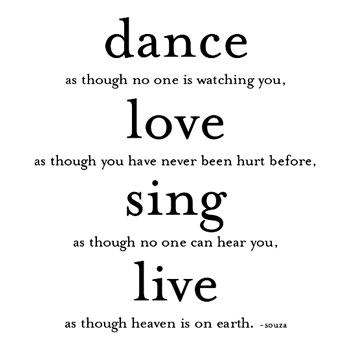The image features a motivational message centered against a stark white background, with all text in black lowercase letters. At the top, the large word "dance" is prominent, followed by the phrase "as though no one is watching you" in smaller text beneath it. Below that, the large word "love" stands out, with the accompanying smaller text "as though you have never been hurt before." Continuing the pattern, the large word "sing" is displayed, under which reads "as though no one can hear you" in smaller letters. Finally, the word "live" appears in large text, followed by "as though heaven is on earth." The text is centered within the image, consuming the majority of the space. At the bottom, the author is identified in small, hyphenated text as "S-O-U-Z-A." The entire composition is designed to convey a heartfelt, inspirational message.